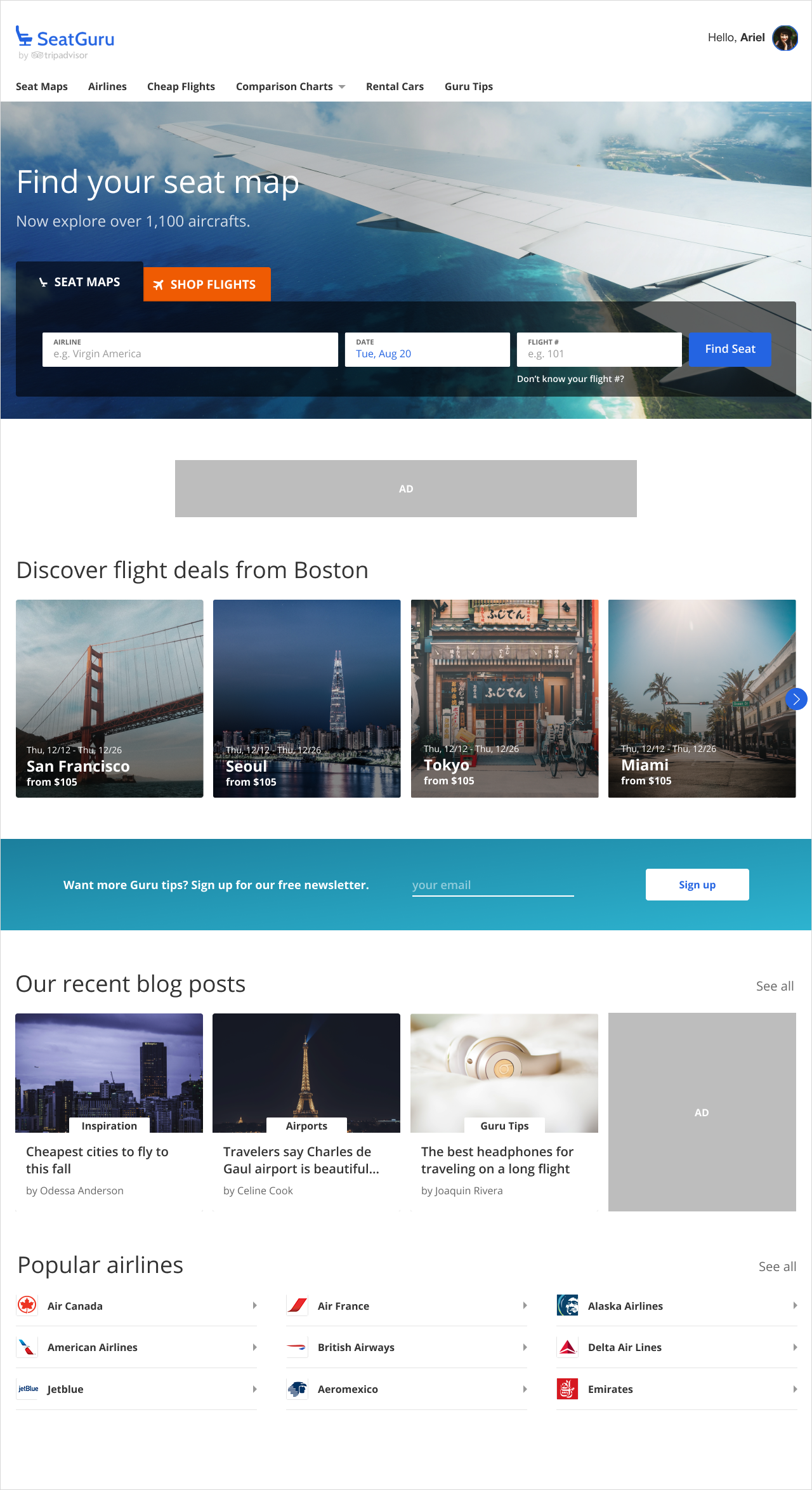This image displays the homepage of the SeatGuru website, a platform dedicated to helping travelers find detailed seat maps for over 1,000 airlines. At the top, it features a navigational section with tabs labeled "SeatMaps" and "Show Flights," which users can toggle between to explore various options. 

Prominently positioned on the page is a search bar divided into three fields labeled "Airline," "Date," and "Flight Number," allowing users to enter their travel details to retrieve specific seat maps. Directly below this search function, there's a button labeled "Find Seat Map," encouraging users to initiate their search.

Adjacent to the primary content, there is an advertisement box, followed by a section titled "Discover Flight Deals from Boston," which highlights promotional flight offers. This section is divided into four smaller boxes, each showcasing different destinations based on the originating city of Boston. 

Overall, this well-organized layout aims to provide users with a seamless experience in locating and understanding their seating options on various flights while also offering travel deals and advertisements.